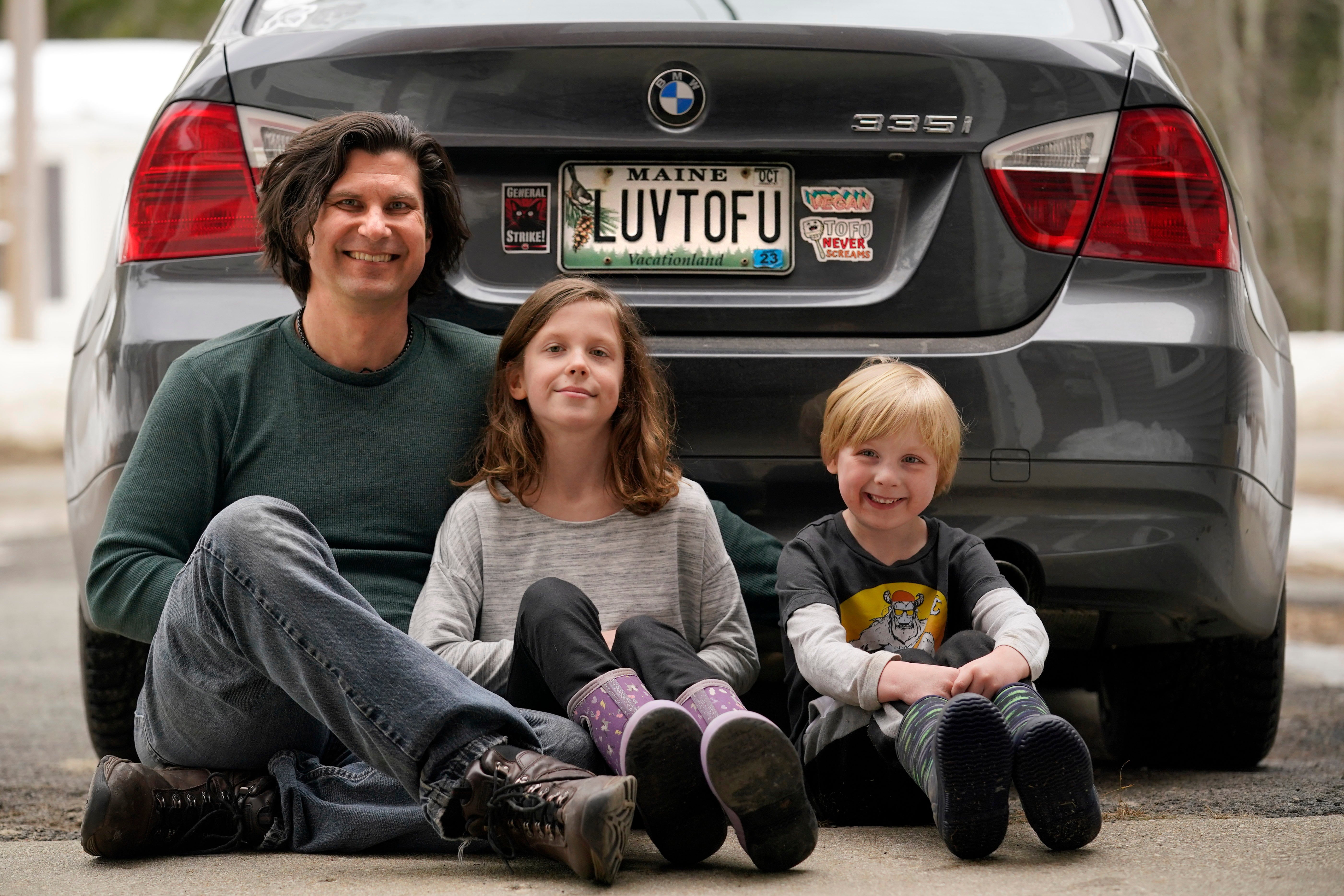A contemporary photograph captures a joyful family moment with a man and two children sitting on the pavement behind their car, a Mercedes Benz 335SI. The vehicle, featuring a Maine license plate that reads "LUV-TOFU," is parked outside with a blurred scenic background. The man, likely the father, has dark black, chin-length hair and a big smile. He's dressed in a hunter green shirt, blue jeans, and work boots. He lovingly has his arms around his two kids. To his right, a little girl with light brown shoulder-length hair, wearing a gray shirt, black pants, and purple rain boots with hearts, smiles softly with her lips closed. On the other side, his young son, with blonde hair and a radiant smile, dons a green and gray shirt, along with black boots. The family's close and cheerful demeanor, highlighted by their bright smiles and relaxed posture, conveys a sense of warmth and happiness.